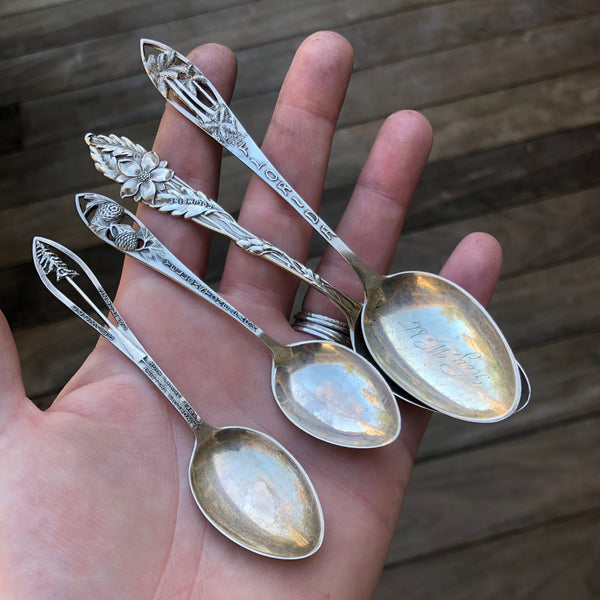The photograph captures a close-up of a left hand outstretched above a background of brown wooden slats. The palm of the hand cradles four antique, tarnished silver spoons, likely collectible items. Three of the spoons are aligned in a row, while the fourth spoon overlaps the third, with the rounded portions of the spoons oriented toward the pinky finger. Each spoon features an ornate handle with distinct designs: one boasts palm trees and the word "Florida," another showcases flowers and leaves, the third depicts pine cones and is the smallest with "Yellowstone Park" engraved on it, and the fourth exhibits a pine tree with additional script on its hollowed-out handle. A silver ring adorns the ring finger of the hand, emphasizing its hold on the delicate, aged treasures.